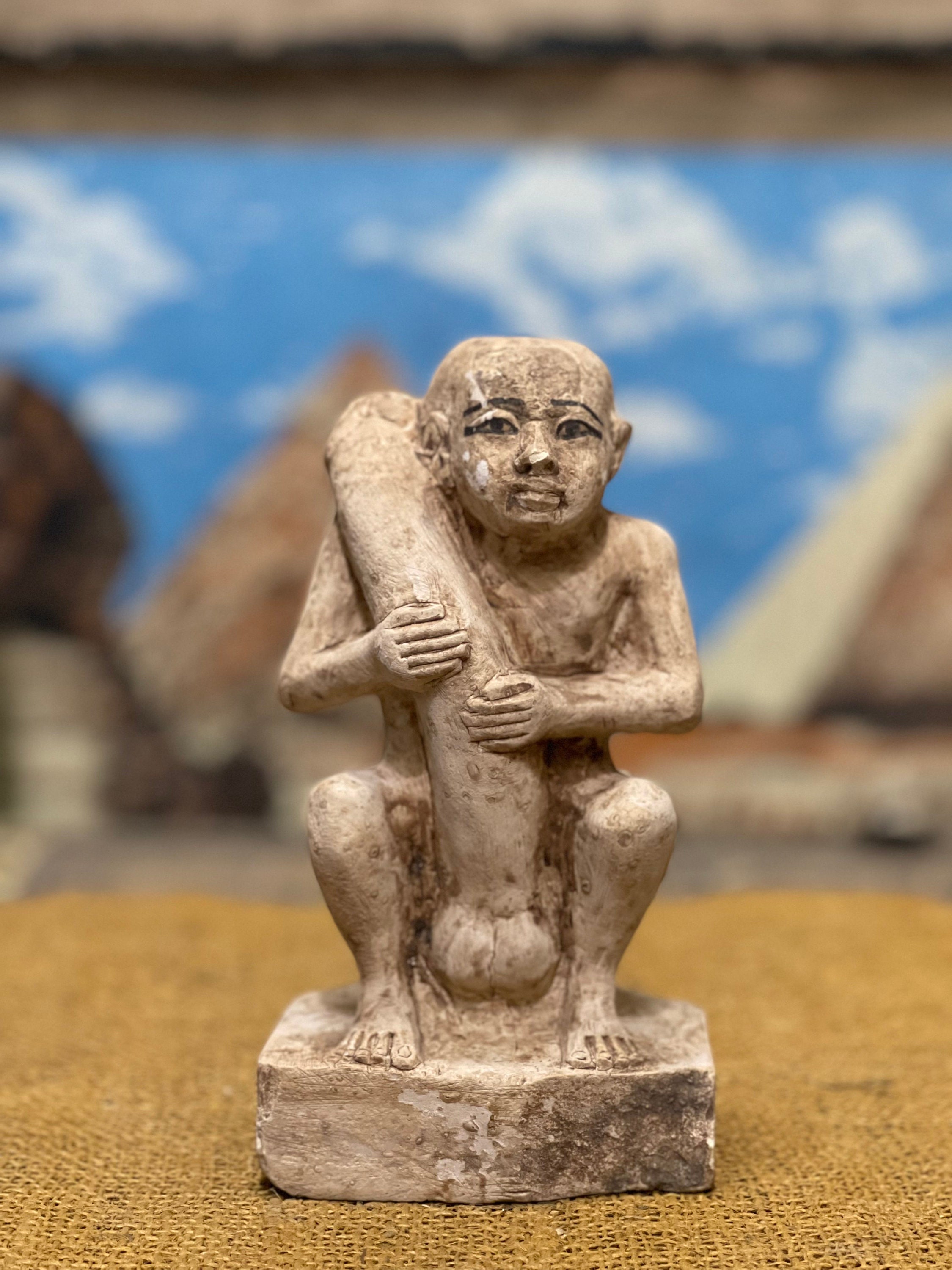This image captures a highly detailed and weathered sculpture of a crouched man, displayed on a woven mat or carpet within an art gallery or museum setting. The small, three-dimensional statue is seemingly carved from stone and possesses a tan hue, with a darker, almost blackish-brown base. The background of the display features blue and white shades, resembling a sky with clouds, along with blurred hints of additional artwork and small stone pyramids.

The intricately crafted figure, which has Asian features, is notable for its bald head, square facial structure, and prominent black eyebrows and eyes. The man is depicted in a naked state, his genitals visibly draped over his shoulder and held in his arms, making the sculpture both provocative and arresting. His large, flat nose and distinct lack of expression add to the statue's enigmatic and ancient allure. The craftsmanship highlights fine details, such as his clearly defined toes and fingers, contributing to the overall impression of an antiquated and exquisite piece of art.